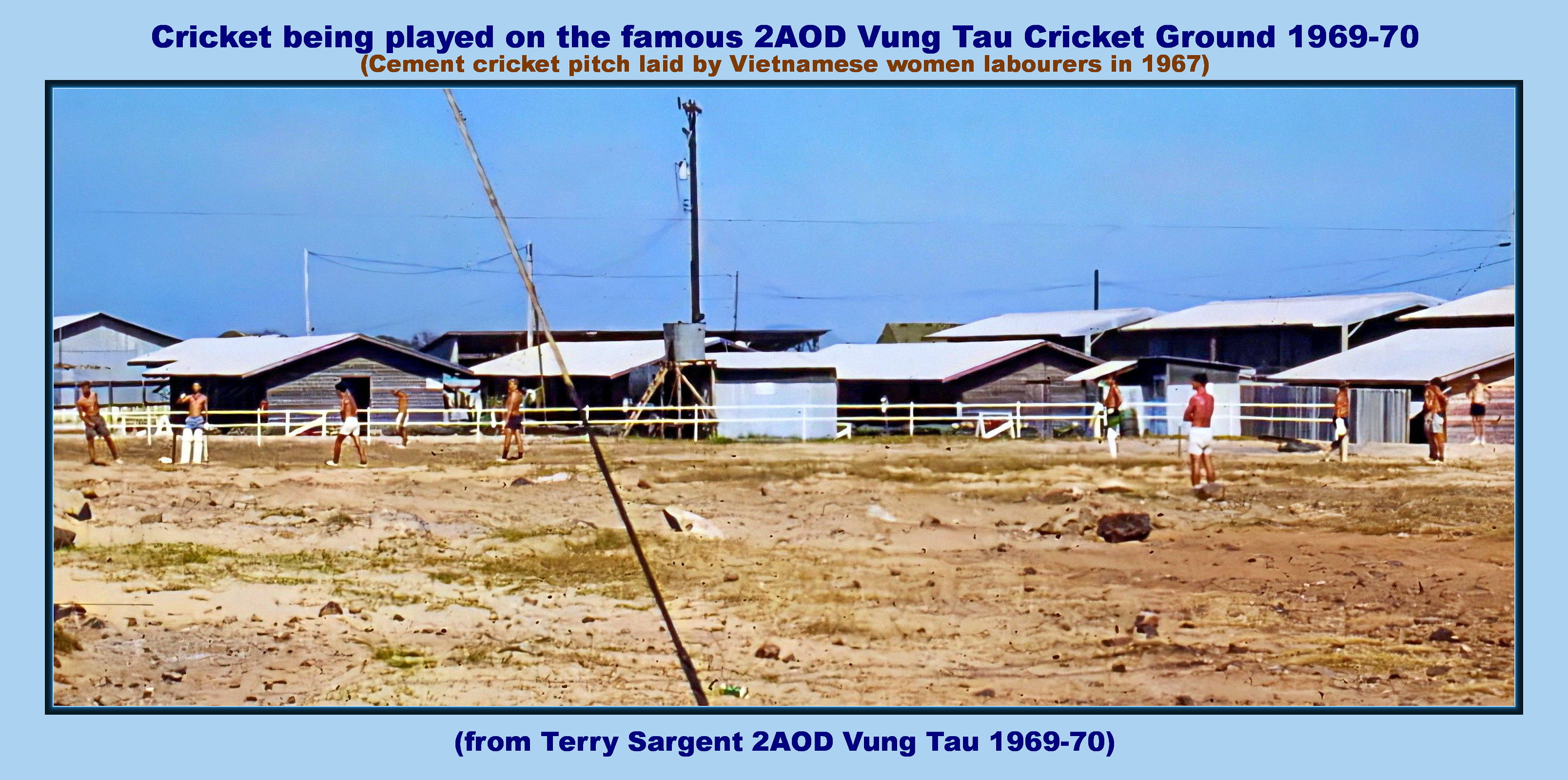The horizontally aligned, rectangular color photograph inset into a larger light blue background captures a daytime scene of cricket being played on a dirty, partially overgrown, and rocky dirt field. The photograph, portraying ten shirtless men in white shorts standing still, is framed by a light blue border with dark blue and red text. The headline reads, "Cricket being played on the famous 2AOD Vung Tau Cricket Ground, 1969-70," followed by a red subhead in parentheses, "Cement cricket pitch laid by Vietnamese women laborers in 1967."  The bottom caption in dark blue reads, "(from Terry Sargent, 2AOD Vung Tau, 1969-70)." The scene includes small, low, single-story wooden buildings with white roofs and a telephone pole with wires running across the background under a clear blue sky. A white fence demarcates the playing area. The image combines photographic realism with graphic design elements, emphasizing both the sport and its historical context.